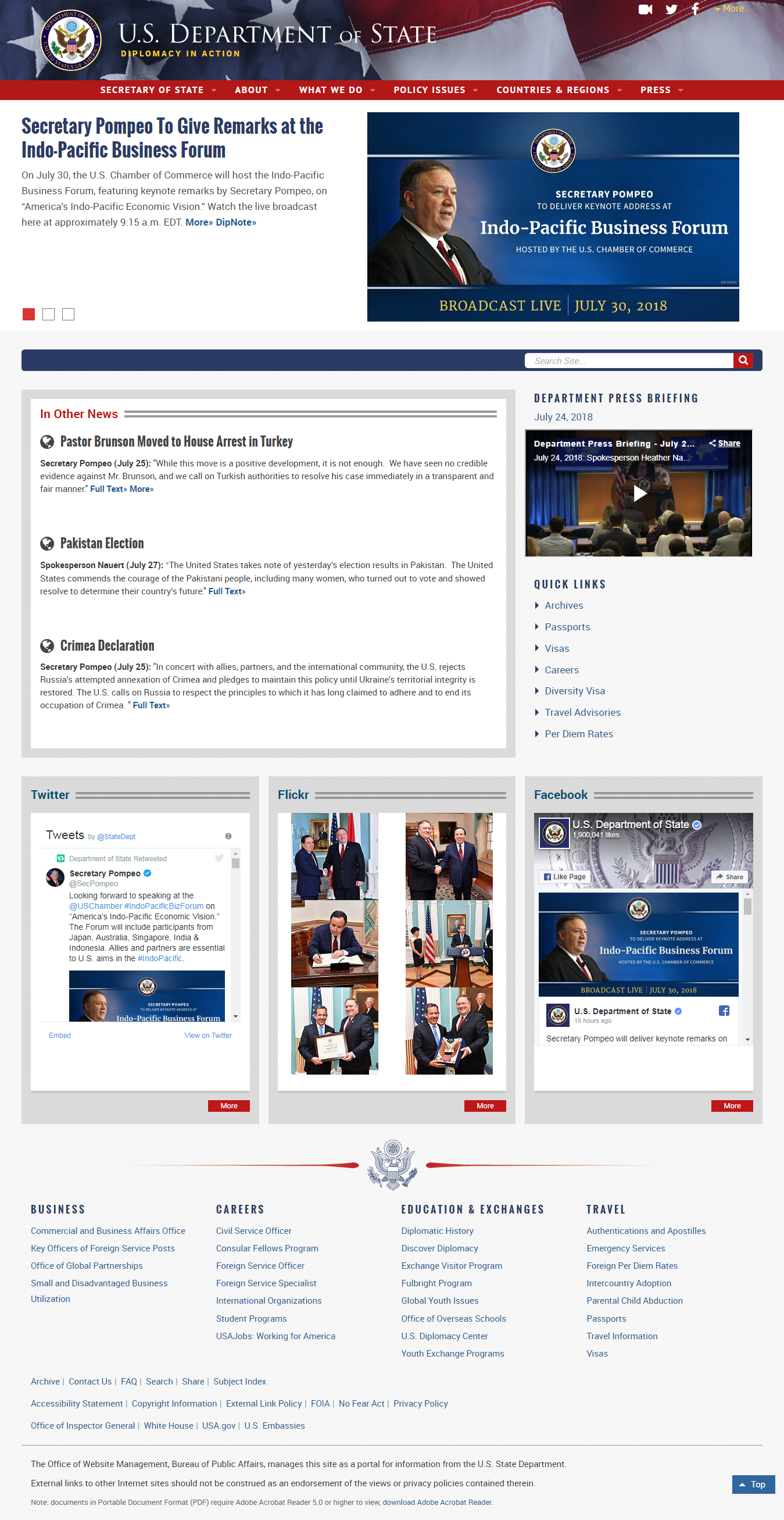Screenshot of the U.S. Department of State Website

The screenshot showcases the official U.S. Department of State website with a prominent red, white, and blue theme. The top of the page features a border displaying the U.S. Department of State logo in the center, which includes an eagle emblem surrounded by stars and stripes that resemble the American flag. Beneath the header, a red navigation bar provides clickable options such as "Secretary of State," "About," "What We Do," "Policy Issues," "Countries and Regions," and "Press."

Central to the page, there's a headline article titled "Secretary Pompeo to Give Remarks at the Indo-Pacific Business Forum." Adjacent to this headline on the right, is an image of Secretary Pompeo. He is depicted in profile, facing to the right, dressed in a suit with a red tie and standing before a blue background.

Below the main content area, a blue bar contains a search box with a magnifying glass icon for easy navigation. Further down, additional sections highlight various news topics, such as the "Pakistan Election" and "Crimea Declaration," alongside a department press briefing.

At the bottom of the screenshot, there are links to the U.S. Department of State's social media profiles, including Twitter, Flickr, and Facebook, signaling available online resources and updates.